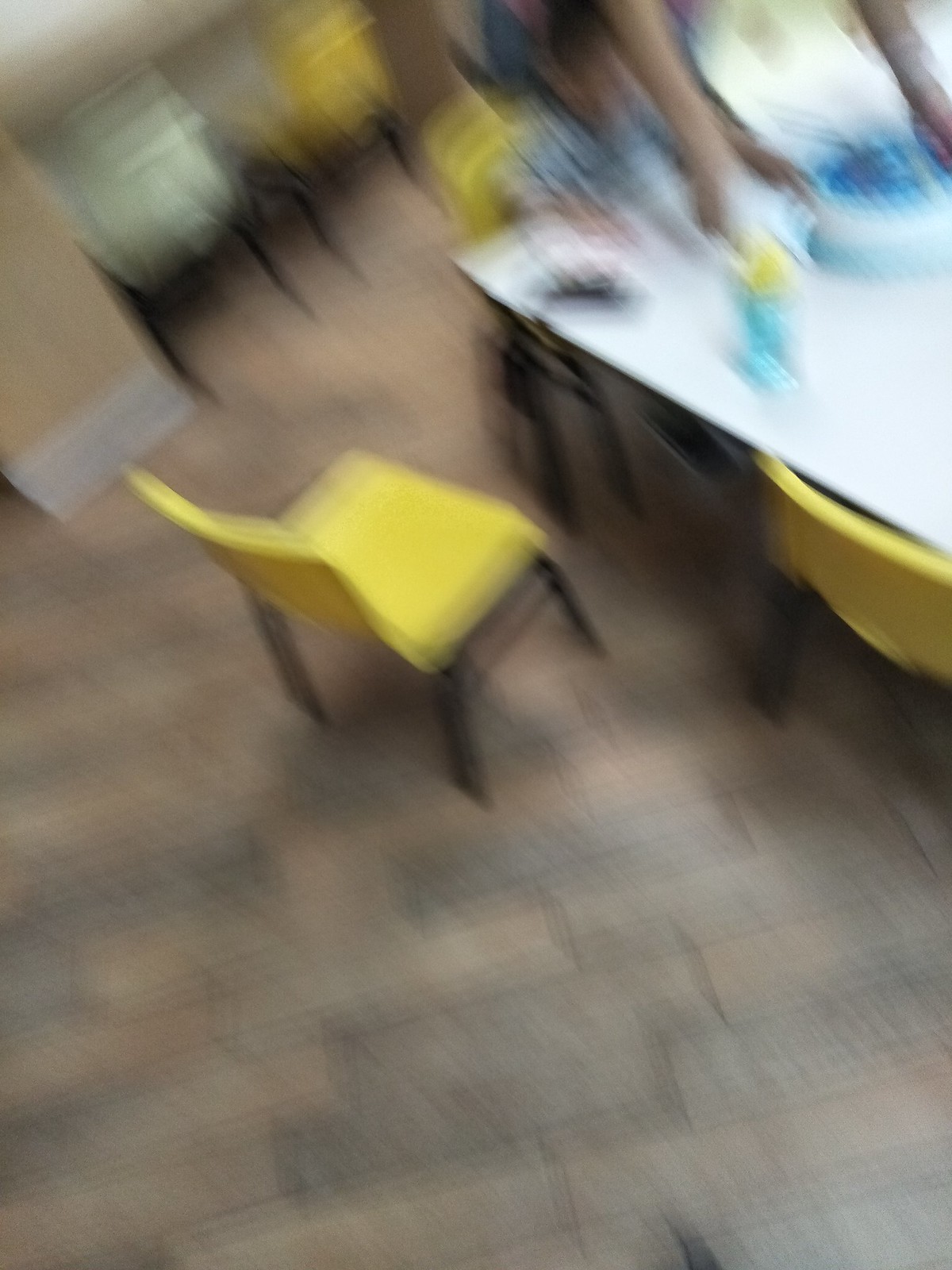In a brightly lit classroom designed for young children, evident from the low table and small chairs arranged around it, a scene unfolds that captures a poignant moment. The classroom, possibly for preschoolers or kindergartners, exudes an air of excitement, although not perfectly mirrored by all its occupants. On the white-surfaced table, a beautifully decorated cake adorned with white and blue frosting sits at the center of attention. This cake, likely intended for a birthday celebration, is being carefully placed on the table by a pair of adult hands just entering the frame from above. Beneath these hands, a small boy sits at the table, his expression hinting at distress or unhappiness. His presence brings a layer of contrast to the otherwise festive setting, suggesting that despite the surrounding festive atmosphere, not everything is as cheerful as it seems for the young boy. The entire scene speaks to the complexity of emotions that can exist even amidst celebratory occasions.